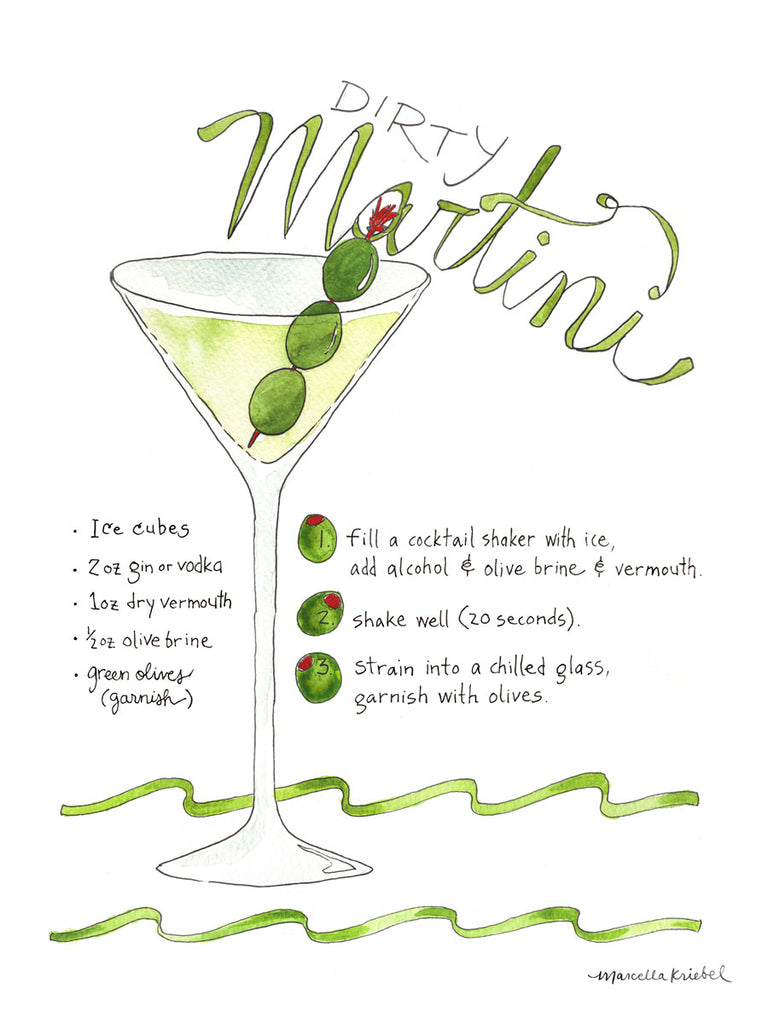This hand-drawn illustration, reminiscent of a cookbook page, vividly details a Dirty Martini recipe. The central image features a clear martini glass filled with vibrant electric green liquid, garnished with a toothpick holding three green olives. The text "Dirty Martini" is prominently displayed at the top right, with "martini" rendered in a ribbon-like pale green script and "dirty" in black, giving it a distinctive and stylish look.

The left side of the illustration lists the ingredients: ice cube, gin or vodka, dry vermouth, olive brine, and green olives. On the right side, three numbered, stuffed olives in red and green provide a step-by-step guide: fill a cocktail shaker with ice, add alcohol, olive brine, and vermouth, shake well for 20 seconds, and strain into a chilled glass before garnishing with olives.

The background is white, highlighting a palette dominated by varying shades of green, accented with strokes of red on the skewered olives. Additional green ribbons, drawn in two bands across the bottom, add a touch of motion and color. The artist's signature resides in the bottom corner, completing this charming, detailed recipe illustration.